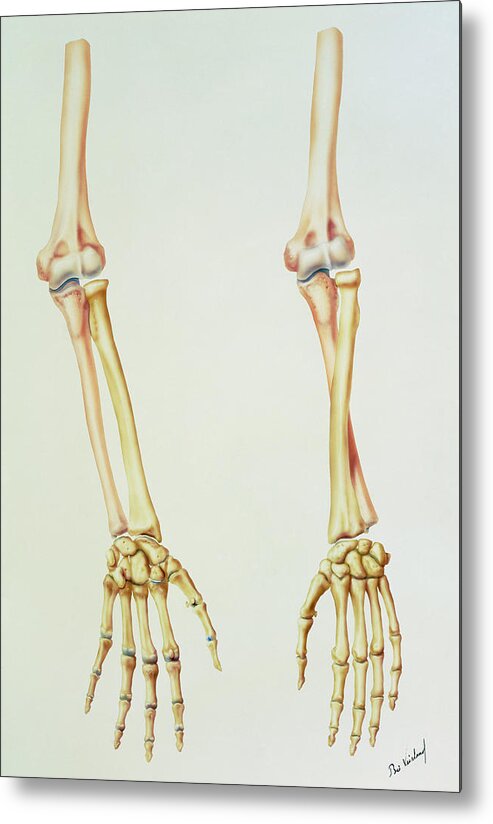This image showcases a detailed, hand-drawn or painted watercolor illustration of two human skeleton arms, each comprising the hand and extending up to the shoulder. Rendered on a white canvas, the bones exhibit a yellowish hue, complemented by brown shadows that intricately reveal the structure of the arms down to the wrists and fingers. The slender bones are accented with delicate shades of pink, red, and green around the joints and tendons. Notably, the arms are depicted with distinct orientations: the left arm's bones run parallel, while the right arm's bones cross at the midpoint. The illustration includes a small, black-inked signature of the artist in the bottom right corner, adding a personal touch to the artwork.